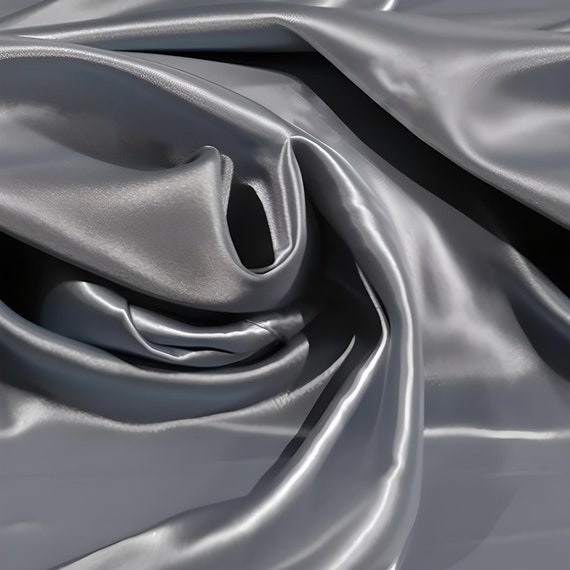The image showcases a glossy, silver-hued silk fabric that is prominently scrunched and twisted, creating intricate folds and shadows. Positioned at an upright angle, the silk cloth forms a soft, almost S-shaped curl in the center of the image, with the deepest folds casting dark, shadowy accents that contrast with the bright, shimmery texture of the material. The silky fabric, possibly featured as part of an advertisement to highlight its luxurious, smooth quality, reveals varying shades of silver as light interacts with its creased, glossy surface. The overall impression is one of elegance and sophistication, with the fabric's lustrous sheen and fluid drape suggesting high-quality silk.